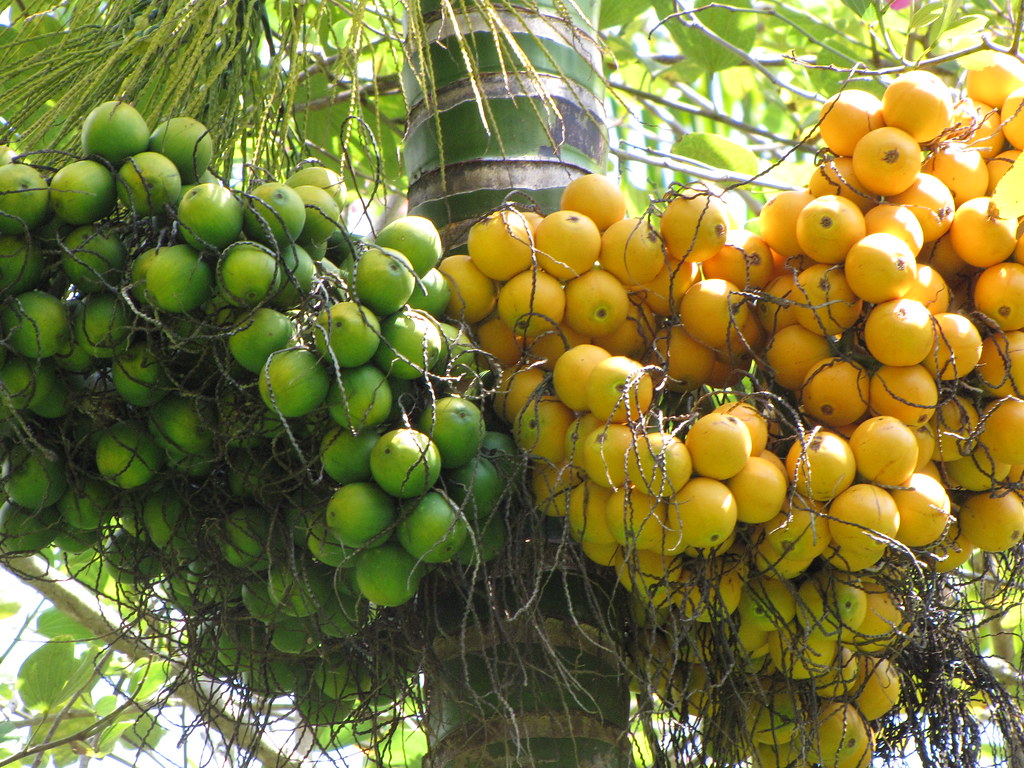The image shows an aerial perspective taken from the ground, capturing a tree with a palm-like base. The trunk features green bands and areas of light gray divots. At the top of the image, there are two distinct clusters of fruit encased in nylon netting: the left cluster contains green, roundish fruits that resemble berries or potentially olives, while the right cluster has yellow fruits, possibly yellow beans or another type of berry. The yellow fruits dominate the scene, extending further downward and filling more of the view compared to the green fruits. The fruits are wrapped around nylon netting and appear to be attached to the trunk of the tree. The daylight reveals sunlight filtering through the foliage, illuminating the greenery in the background. The trunk, which is also partially wrapped in green paper, appears blackish where it lacks light. To the sides and background of the main structure, tree branches and large leaves are visible, contributing to the lush, green scenery.